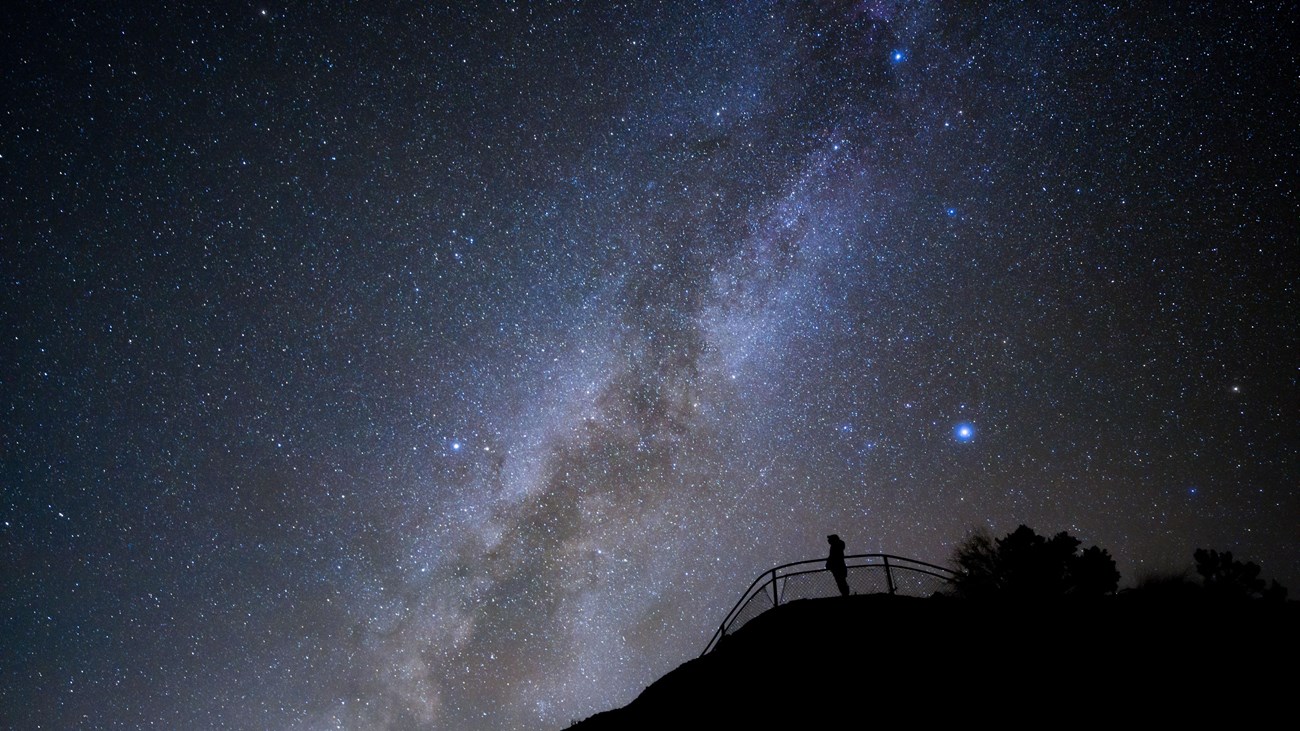In the image, a silhouetted figure, possibly a woman in a parka, stands on the edge of a mountain at a scenic overlook, gazing up at a breathtaking night sky. A metal railing with webbing at the bottom prevents anyone from venturing too close to the edge. Some bushes are visible behind the person, adding depth to the scene. The sky above is filled with a myriad of stars, with a striking galaxy-like formation dominating the center. This celestial feature begins with a gray band that transitions into a lighter white hue, then shifts into soft purples as it extends outward, becoming darker at the edges. On the right side, three bright blue lights align vertically, with the middle one slightly dimmer, and the top one encircled by a dark blue ring. The left side of the sky appears darker, dotted with numerous tiny stars in shades of white and blue. The photograph, possibly enhanced or generated digitally, captures the awe-inspiring beauty of the night sky from a lower vantage point, looking up at the figure standing above.